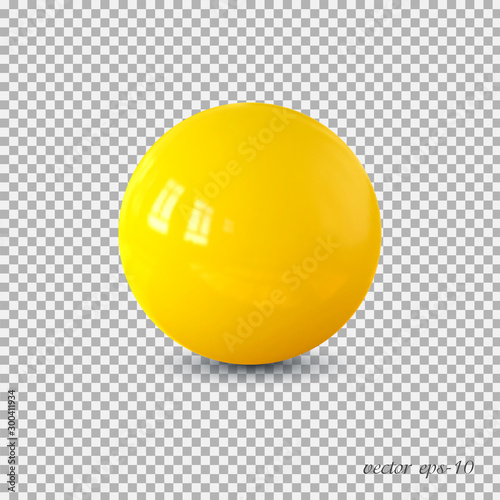The image features a realistic-looking yellow sphere situated prominently in the center. The sphere captures light reflecting from what appears to be windows, creating two bright white spots on its surface. Subtle shadows beneath the sphere enhance its three-dimensional, lifelike quality. The entire background is a compact checkerboard pattern of alternating white and gray squares, indicative of transparency in digital imaging. Overlaying the sphere are two watermarks that read "Adobe Stock." Additionally, the bottom left corner displays the text "Adobe Stock #300411934" in vertical black letters, while the bottom right corner reads "Vector EPS-10" in horizontal black letters.